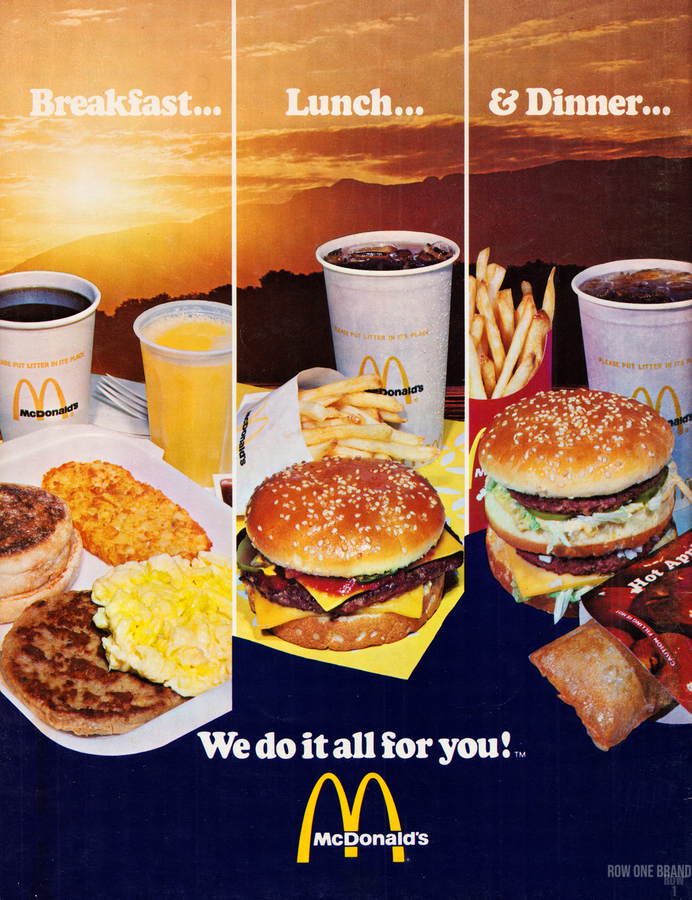The image is an advertisement for McDonald's featuring breakfast, lunch, and dinner options, divided into three sections. On the left, the "Breakfast" section is highlighted by a bright orange sunrise in the background. This section includes a yellow cup filled with dark black coffee and a plastic cup of orange juice. There's a white tray with an orange-colored omelet, cooked sausages with blackened spots, scrambled eggs, hash browns, and a biscuit.

In the middle, the "Lunch" section features a backdrop of a mountain range with orange-hued clouds. A classic hamburger with a seeded brown bun, black meat, and yellow cheese is prominently displayed. A white bag with golden french fries and a white cup filled with a dark soda, ice chips floating to the top, accompany the burger.

The "Dinner" section, located on the right, has the text beside an ampersand symbol. This part of the poster includes a double hamburger with white sesame seeds on the bun and dark brown meat inside. Behind the burger is a red box of yellow french fries and a white cup filled with dark soda and ice. Additionally, a slice of light brown cake with glaze is visible in a red package.

At the bottom of the image, in white text, it says "We do it all for you." Beneath this slogan is the iconic yellow McDonald’s "M" logo, followed by the text "McDonald's." In the bottom right corner, light gray text indicates "Row 1 brand." The background of this lower section is a dark black color.